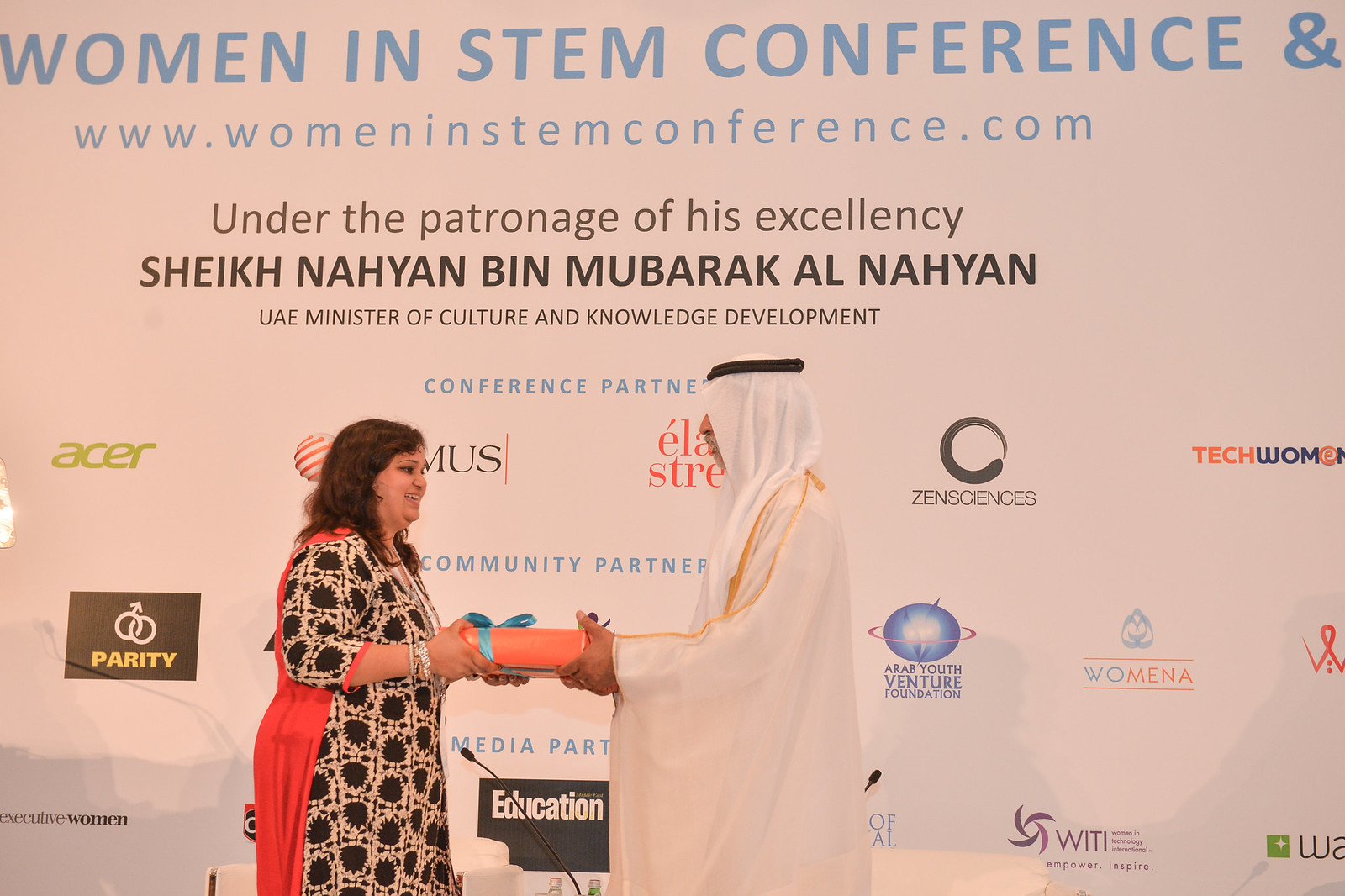The photograph showcases a moment at the Women in STEM Conference, as indicated by the large backdrop which reads, "Women in STEM Conference, www.womeninstemconference.com." The event is held under the patronage of His Excellency Sheikh Nahyan Bin Mubarak Al Nahyan, UAE Minister of Culture and Knowledge Development, with various sponsors displayed prominently, including Acer.

In the image, a woman on the left is receiving an award from a person on the right, who appears to be a man. The man is dressed in an all-white gown with a covered head, secured by a black bandana. He is handing the woman a rolled-up piece of orange paper adorned with a blue bow. The woman is smiling graciously as she accepts the award, dressed in a distinctive outfit with a black and white front and an orange back. The scene is vibrant and colorful, highlighting the celebratory and prestigious nature of the event.